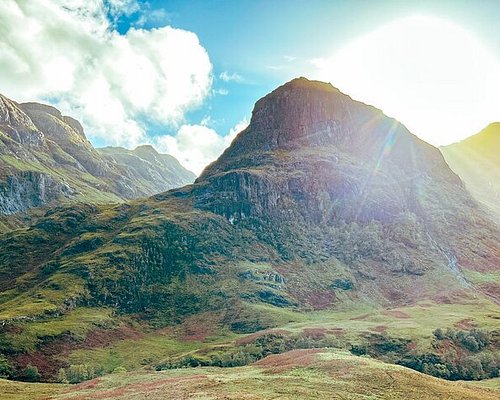The image captures a clear and vivid daytime scene of a mountain range under a bright blue sky. The mountains, primarily composed of dark brown to reddish exposed rock, feature a somewhat stubby, plateau-like appearance rather than sharp peaks. In the foreground, the rocky terrain gradually transitions into a grassy, mossy, and bush-covered landscape, with green hues becoming more prominent towards the base of the mountains. To the left side of the image, puffy white clouds dot the sky, while on the top right, the sun emits radiant beams, creating a slight haze and a faint rainbow refraction effect. There are no people, words, or numbers in the image, allowing the natural beauty of the outdoor landscape to be the focal point.